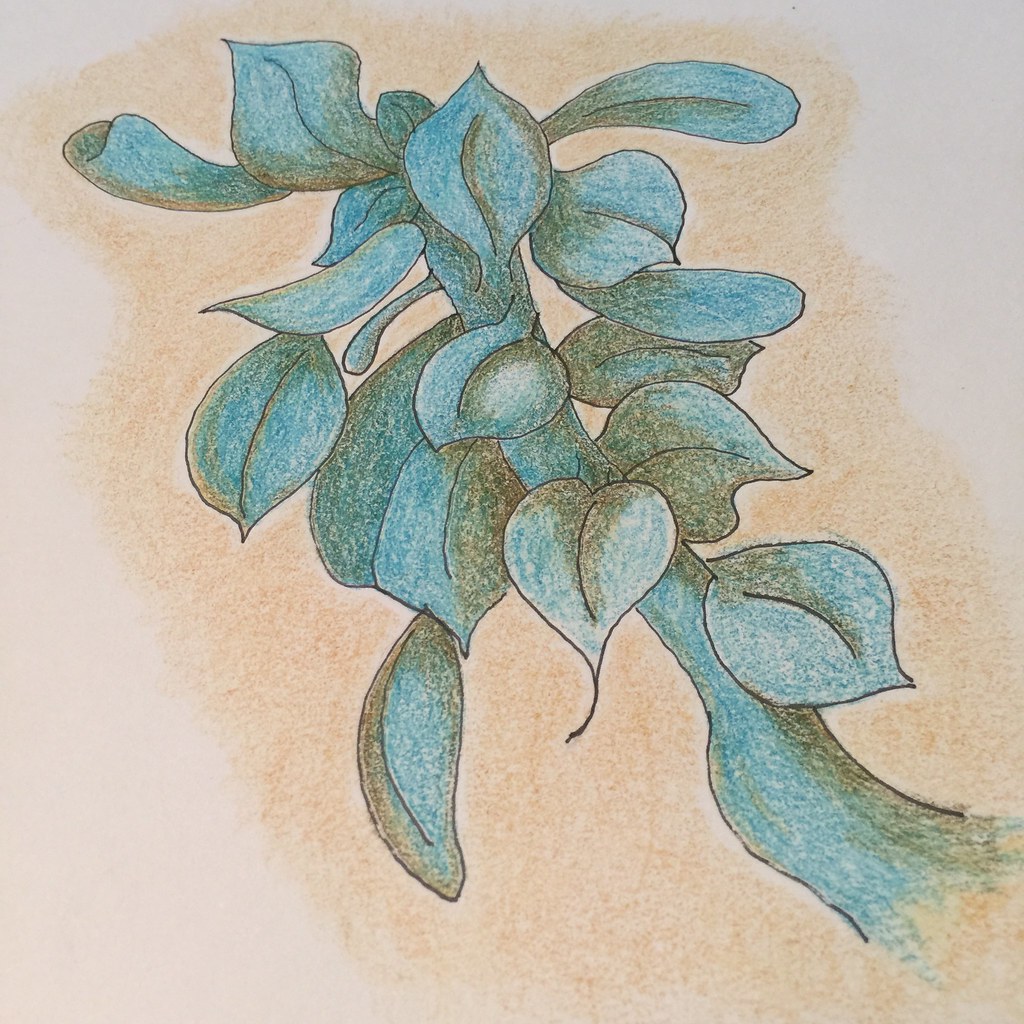The image features a white paper background adorned with a detailed crayon drawing of a blue plant. The plant's stem and leaves are uniformly blue, but the leaves also feature areas of black shading that adds depth and dimension. The stem gracefully curves upward, culminating in over ten leaves that fan out in various directions. Each leaf displays intricate black lines and slight speckling, allowing glimpses of the white paper beneath, which enhances the crayon-like texture of the drawing. Surrounding the blue plant, there are subtle hints of brown and white, which provide a contrasting backdrop to the vibrant blue. The black shading on the tips of some leaves adds an additional layer of complexity and realism to the artwork.